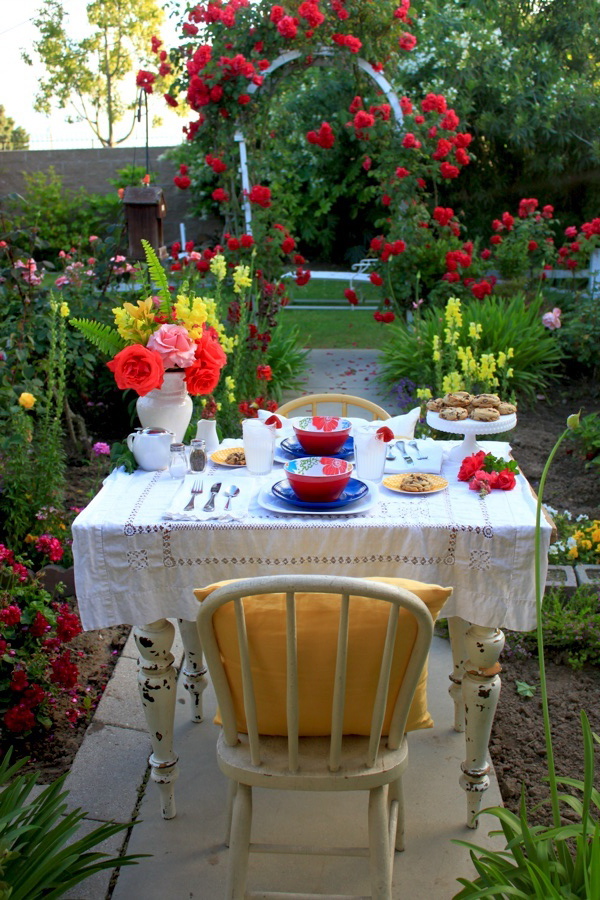This vibrant, color photograph captures a serene outdoor setting in a lush flower garden. Central to the scene is a quaint, white, rustic table with chipped, worn legs, standing on a concrete walkway. The table, adorned with a white tablecloth, features a setting for two, including white underplates, blue smaller plates, and red bowls. Each place setting is completed with forks, knives, and spoons. Among the table’s charming details are a pair of salt and pepper shakers, a teapot, and a creamer pot. A plate of chocolate chip cookies and a white vase brimming with blooming red and pink roses adorn the table, along with two glasses of water and scattered red flower petals.

Flanking the table are old white chairs, each softened with a yellow throw pillow. The surrounding garden bustles with life, featuring vibrant red and yellow roses, pink flowers, white and yellow blooms, green leaves, ferns, various bushes, and trees. An arched trellis with red flowering plants stands nearby, adding a touch of elegance to the scene. The distant backdrop reveals a glimpse of a house, completing this picturesque setting.